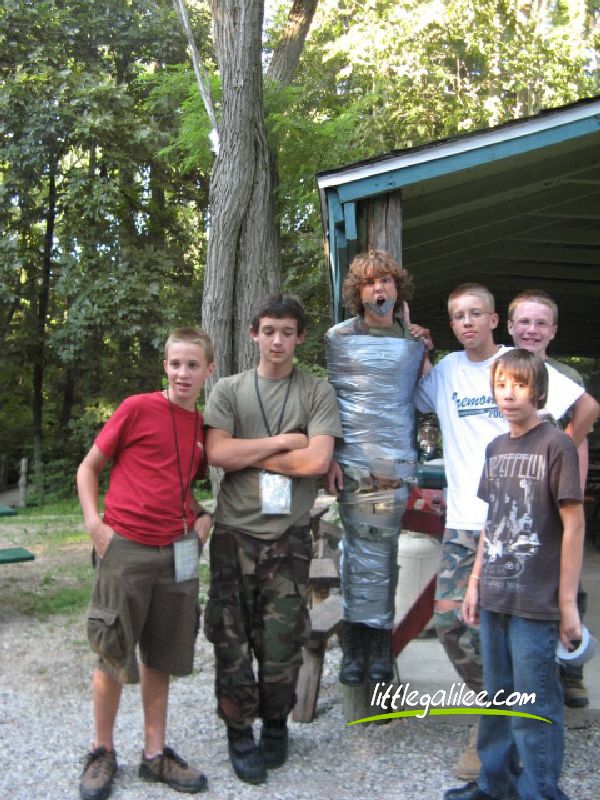In this image, six teenage boys of European descent are posed outdoors, standing on what appears to be a gravel driveway or lawn area with a wooded background. Centered in the group is a boy with shaggy, curly hair who has been duct-taped to a pole from his ankles to his shoulders, with additional tape over his mouth, partially open as if he is yelling. Two boys to his left wear lanyards: one has a red shirt and green shorts, while the other wears camouflage pants and a green shirt with crossed arms. On the right side, the boy closest to the front is the shortest, sporting short hair, a Led Zeppelin shirt, and jeans, while two other boys, both with very short hair and glasses, stand behind him; the one in the white shirt is holding the shoulder of the taped boy, and the other, partially covered, wears a greenish shirt. In the background, there's a large tree trunk and a man-made shelter, likely a garage or roof. The image features a littlegalilee.com watermark at the bottom, suggesting the photo was taken at a camp.